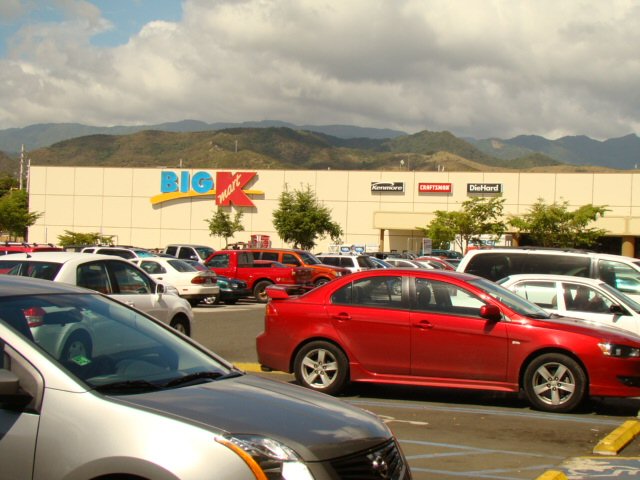The image features a large white Kmart building with a distinctly squared facade and a prominent "Big K" sign in blue and red letters, underlined in yellow. Above the store, the sky is mostly filled with dark gray and white clouds, suggesting an imminent rainy day, although a hint of blue sky is visible in the top right corner. In the distant background, there are faintly visible mountains and green, hilly terrain. 

In front of the store entrance are three noticeable signs: "Kenmore," "Craftsman," and "Die Hard." Several small trees are positioned near the entrance and scattered around, including a bushy tree on the left end of the building. 

The parking lot is bustling with vehicles. Notable cars include a close-up silver car, a white car driving through the lot, and several parked vehicles: a red car, a white car, a white minivan, and some additional red trucks and white cars further in the background. The image captures the busy atmosphere outside the Kmart store on a cloudy day with looming rain.